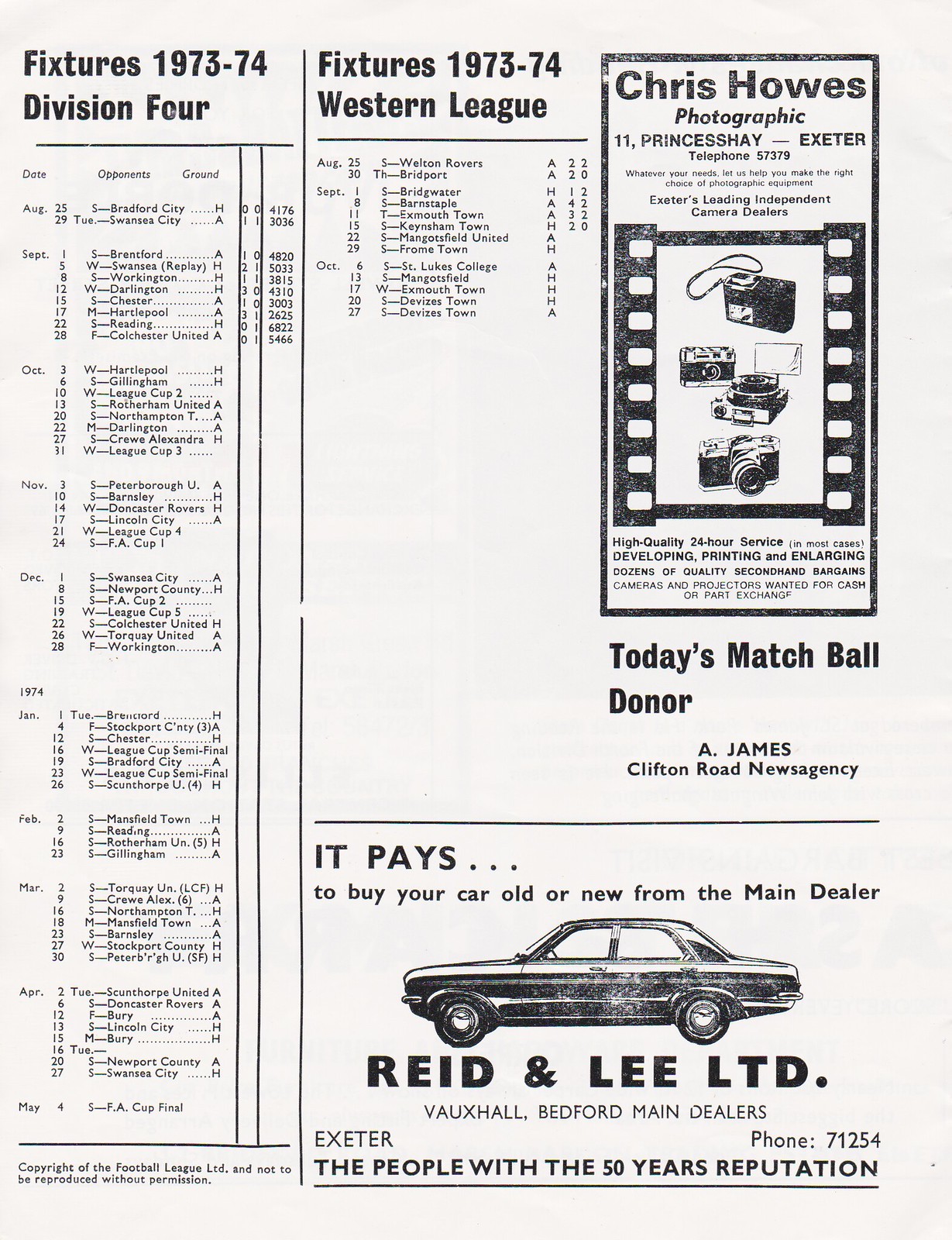The image appears to be a black and white scan of a vintage page, likely from a newspaper or magazine, predominantly featuring sports fixtures and advertisements. The left column is titled "Fixtures 1973-74, Division 4," detailing a list organized by months, including dates, opponents, and grounds for a soccer league. Adjacent to it, another column titled "Fixtures 1973-74, Western League" contains a similar breakdown of dates, opponents, and grounds. Below these sections, there's an advertisement for "Chris House Photographic, 11, Prince, Hey, Exeter," featuring illustrations of cameras and a contact telephone number. Additionally, there's a note stating "Today's Matchball Donor, a James Clifton Road News Agency." At the very bottom of the page, a car advertisement showcases a sedan with the tagline, "It pays to buy your car old or new from the main dealer, Reed & Lee LTD."